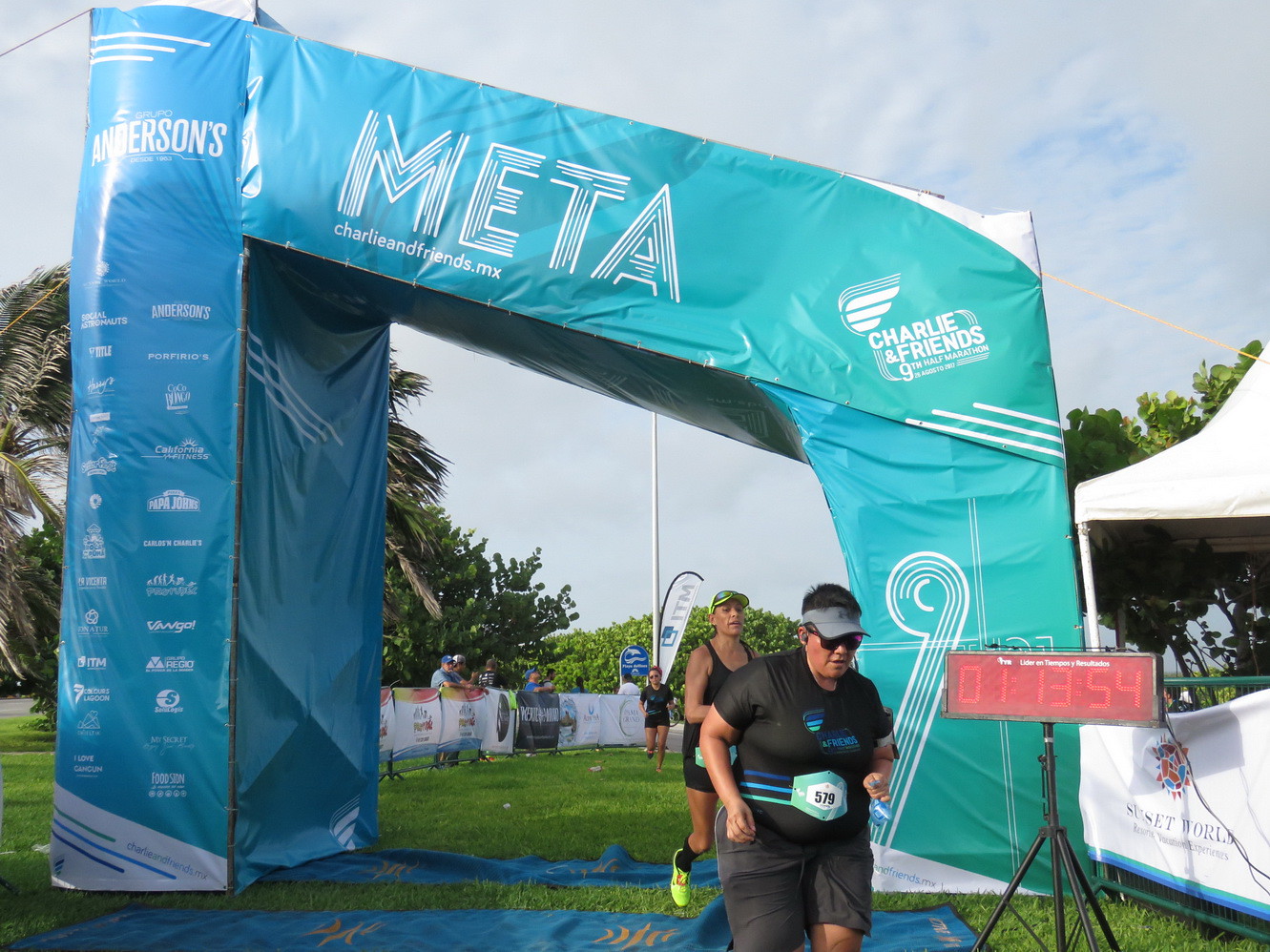The photo captures the dynamic finish line of a marathon. The focal point is a slightly off-centered inflatable arch, taller on the left side and lower on the right side, adorned in blue and turquoise hues. Prominently featured is the leading runner, wearing bib number 579, donning a black outfit, a visor hat, and sunglasses. She has just crossed under the arch, followed closely by a second runner who has recently finished and a third runner visible in the distance approaching the arch. To the right, a red digital clock displays the race time as 1 hour, 13 minutes, and 54 seconds. Above the arch, a banner reads "meta" and "charlieandfriends.mx," adding context to the marathon scene bustling with competitors.